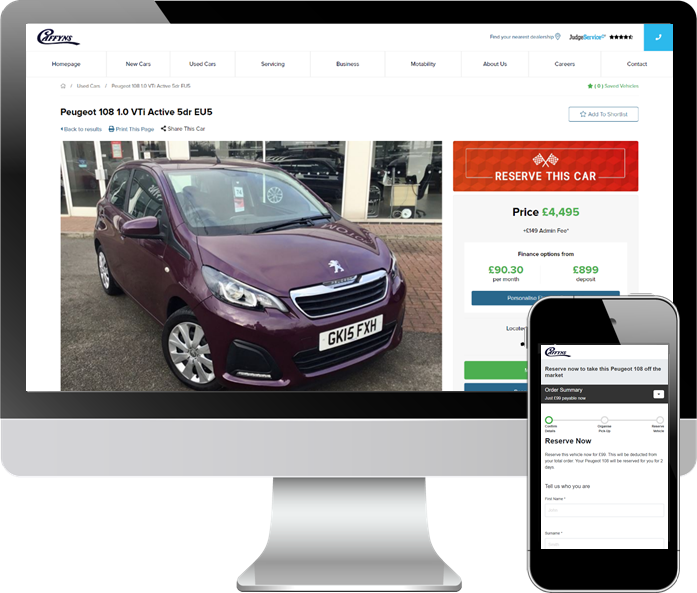The image displays a detailed online car dealership webpage viewed on an iMac. The screen predominantly features black icons and text, along with a variety of colorful elements. At the top of the page, you'll find navigation options labeled "Homepage," "New Cars," "Used Cars," "Servicing," "Business," "Motability," "About Us," "Careers," and "Contact."

In the main section, a blue square icon resembling a phone symbol indicates contact details. Below this, there’s a listing for a used car, specifically a Peugeot 108 with a 1.0 VTI Active engine, identified by its detailed specifications: FTI, DR, EU5.

Accompanying the listing are several actionable buttons: "Purchase All," "Print This Page," "Share This Car," and "Add to Shortlist." An orange rectangle aptly encourages users to "Reserve This Car," pricing it at £4,495. Finance options are available starting from £90.30 per month with the possibility of paying a non-deposit.

The center image of the Peugeot 108 is shown in a distinctive purple color, with the registration number "GK I5 5XH" visible. Below this, there's a note pointing to potential additional features to the right, possibly specifying "some kind of smartphone thing."

The iMac is positioned on a metal stand with a brick-patterned floor underneath, suggesting a modern display area in a dealership or showroom.